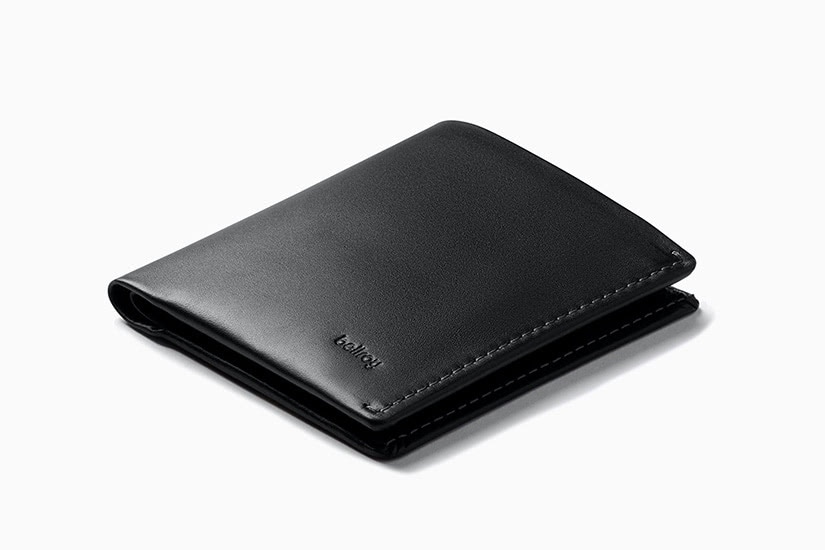This photograph showcases a sleek, black leather bifold wallet set against a nearly pure white backdrop. The wallet displays meticulous craftsmanship with fine, detailed stitching running along the edges. Notably, it features an embossed manufacturer’s logo, "Bellroy," in lowercase letters in the bottom right corner. The wallet appears to be made of high-quality, smooth leather, possibly genuine or synthetic. The lighting in the image creates a subtle, gray drop shadow behind the wallet, which is angled slightly upward to the right, giving it a dynamic appearance against the minimalist background.